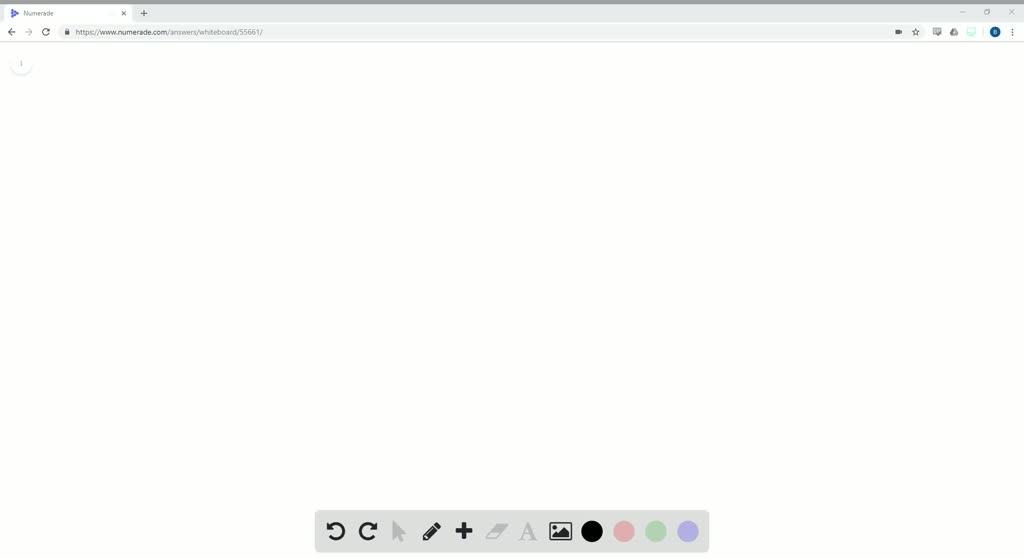The image features a web browser window with a light gray border at the top. The content is incredibly blurry and small, making it difficult to discern specific details. 

In the top section, an address bar is visible with some form of URL inside it, accompanied by various icons to its right. Among these icons are a dark blue circle and a vertical ellipsis. Also present are the standard minimize, maximize, and close (X) buttons.

Below this bar, on a light gray background, a small circle with an indistinguishable icon is positioned at the top left. At the bottom of the window, there is a rectangular gray shape housing several icons and buttons. On the left side of this rectangle is a refresh button, while the right side contains a sequence of icons: a forward button, a pencil icon, a plus icon, a photo icon, a black circle, a pink circle, and a blue circle.